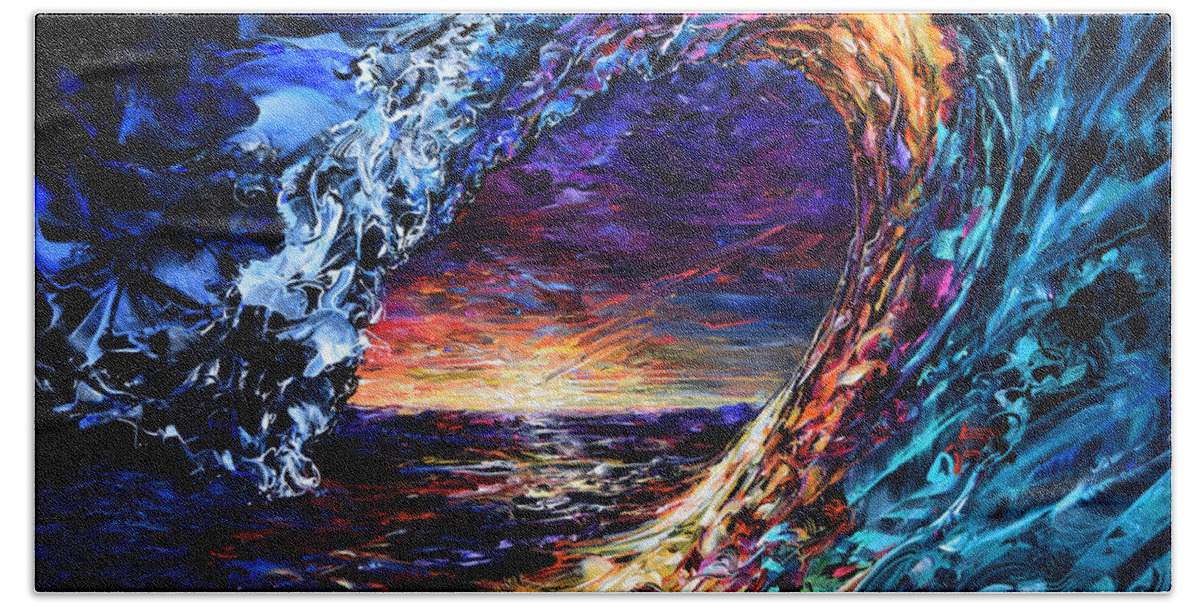This color illustration captures a dramatic seascape at sunset, featuring a dynamic, curling wave. The wave, emerging from the bottom center of the image, arcs around to the right, nearly completing a full loop before crashing down on the left side. The ocean's hues transition from dark blue to purple with red accents where it reflects the sun, which is setting on the horizon about two-thirds down from the top. The wave itself displays a remarkable gradient: aqua on the right with gold at the top, shifting to blue and white foam as it circles back to the left. White foam is visible along the wave's edges, contributing to the turbulent texture. The sky above mirrors the ocean's vibrant palette, with a deep purple at the top, blending into red and yellow near the sea level. Abstract shapes within the wave add an imaginative touch, possibly hinting at faces. The overall style is abstract, showcasing the swirling interplay of light and color in a breathtaking sunset scene.